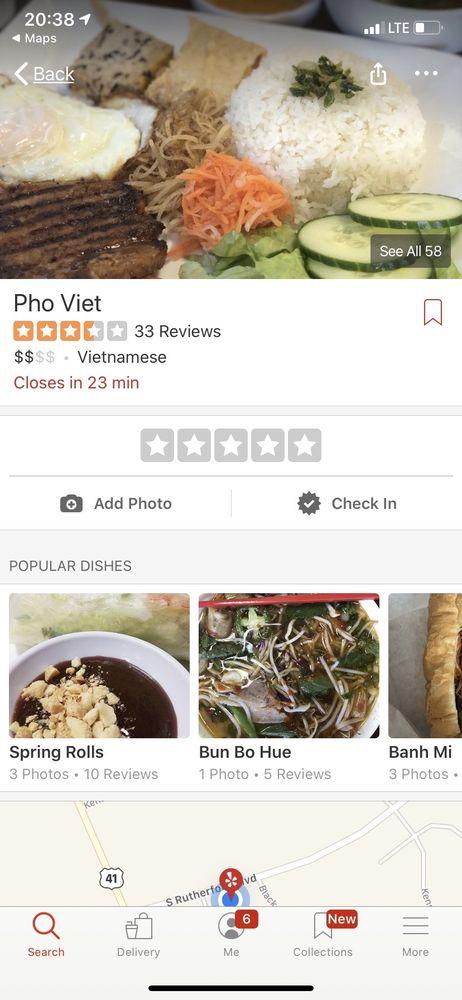The image displays a smartphone screen with a variety of information about a Vietnamese restaurant called "Pho Viet." At the top, the screen shows the current time as 20:38, a signal strength indicator with 3 out of 4 bars, and a battery icon indicating approximately one-third of the battery remaining. 

Below this top information, there are navigation buttons labeled "Back" and "Forward," alongside a download button and an ellipsis menu for additional options.

The central part of the screen features a photo of a dish that includes shredded carrots, rice, cucumber slices, and an over-easy egg. Underneath the photo, the restaurant's name "Pho Viet" is displayed along with a rating of 3.5 stars based on 33 reviews. The text indicates that the restaurant serves Vietnamese cuisine and is closing in 23 minutes.

Further down, there are options to add a photo or check-in at the restaurant. Below these options, a section titled "Popular Dishes" shows three images with descriptions and reviews: 
1. Spring Rolls - 3 photos, 10 reviews 
2. Bun Bo Hue - 1 photo, 5 reviews 
3. Banh Mi - 3 photos

At the bottom of the screen, a map is displayed with a location pin indicating where the business is situated.